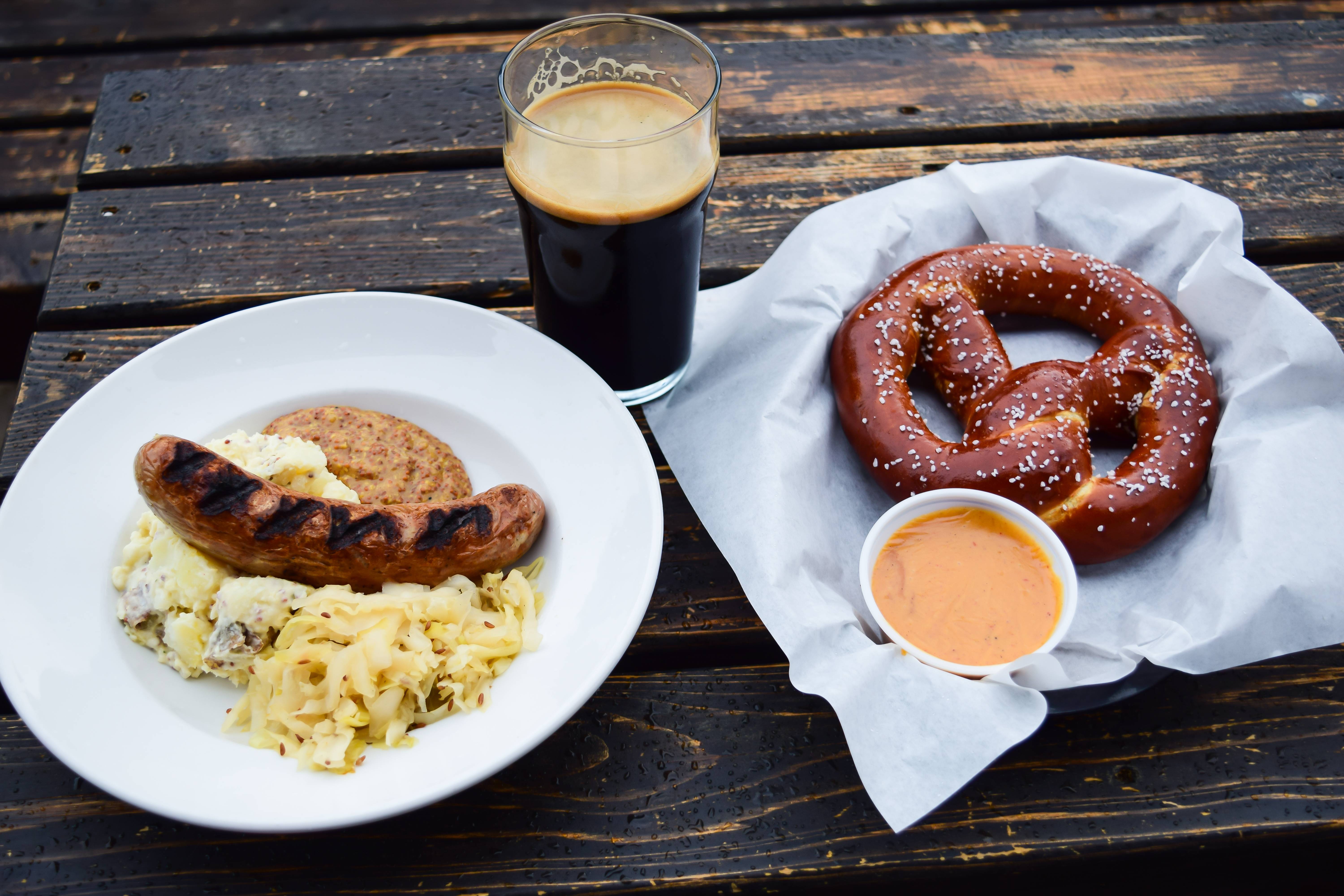The photograph captures a rustic outdoor dining scene, likely at a restaurant or possibly during an Oktoberfest celebration, featuring classic German fare. The setting is a vintage picnic table made of dark-stained wooden slats with lighter wood grain and fading visible, illuminated by sunlight. On the left, a white china dish holds a grilled sausage with char marks, nestled on a bed of mashed potatoes and sauerkraut, accented by a dollop of brown mustard. Adjacent to this is a large, salted pretzel sitting atop white parchment paper inside a basket, accompanied by a white ramekin filled with yellow cheese sauce. In the background, partially consumed, is a pint glass of dark beer, probably a porter or ale, with a tan foam head.